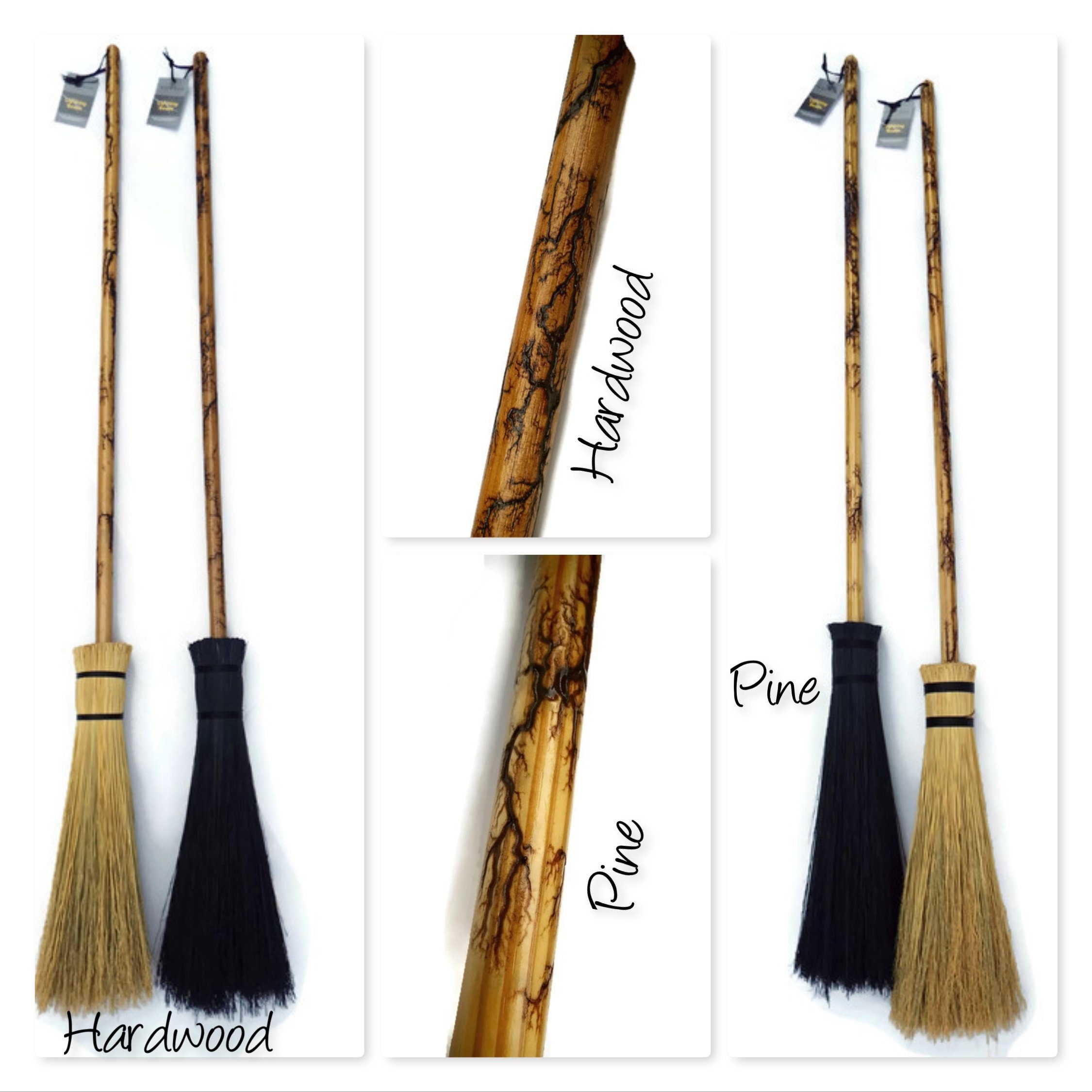This composite image features four handmade brooms, reminiscent of those from witchcraft folklore, likely showcased as a listing for sale, possibly on Etsy. The image is divided into segments: the left side displays two brooms labeled "hardwood"—one with a light, tan color and the other in black. Each broom has a long wooden handle with an etched, lightning-like, tree pattern, adding a rustic and handcrafted charm. In the center, there are close-up shots of the broom handles, further highlighting the intricate designs that resemble the effects of electricity or burning on the wood. On the right, two more brooms labeled "pine" are shown; one black and the other a pale yellowish color, both featuring similar detailed handle patterns as the hardwood brooms. The meticulous craftsmanship and natural aesthetic suggest these brooms could be used as decorative pieces, particularly in a Halloween display.